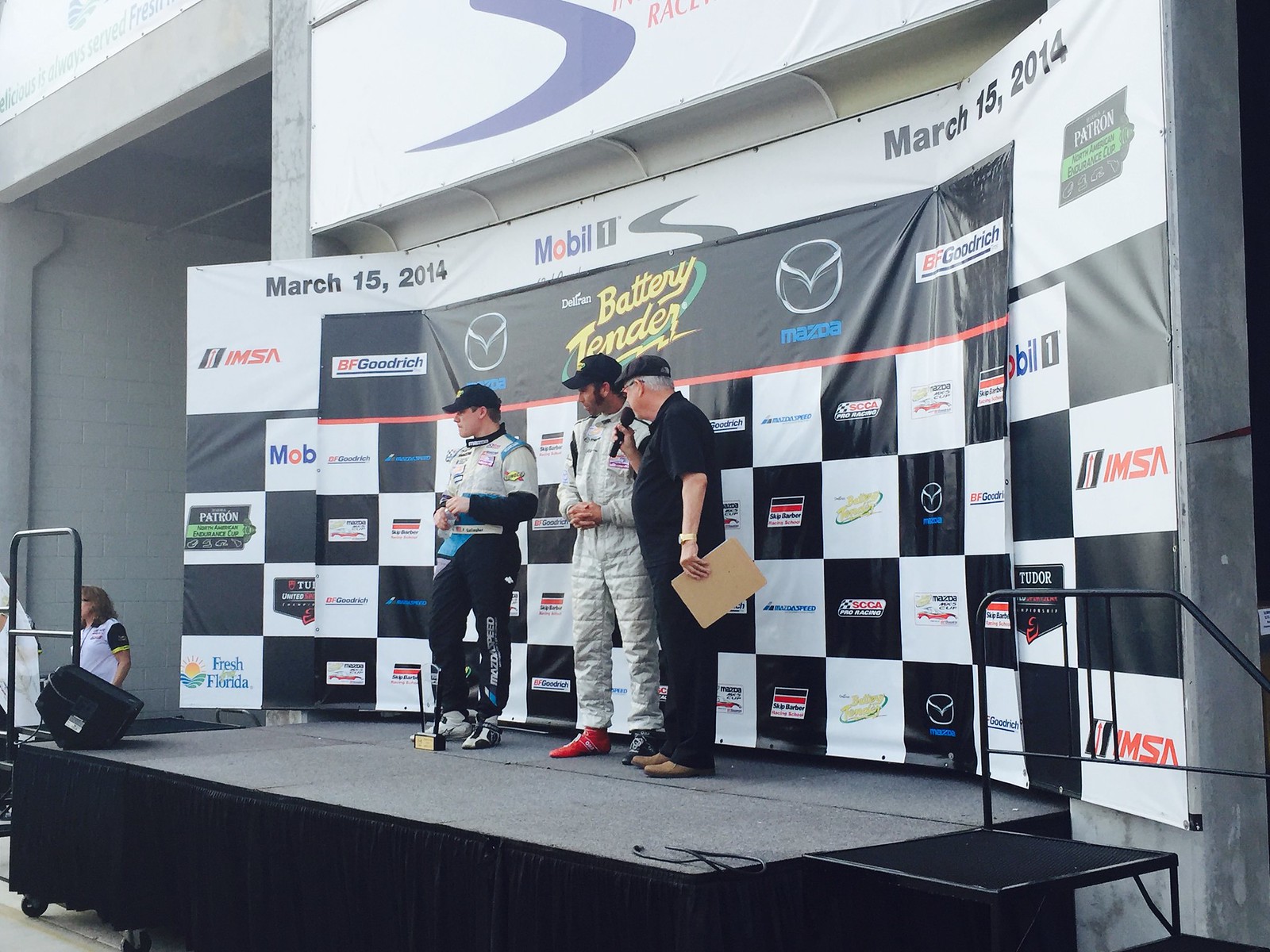The photograph captures an outdoor semi-professional motorsport event stage set up on March 15, 2014. The stage, adorned with a gray carpet top and a black skirt around its perimeter, also features black steps on either side. Three men are standing on this compact stage, indicative of a modest racing event. One man, dressed entirely in black and holding a microphone and a brown notepad, is interviewing two racers. The first racer, positioned in the center, sports a white jumpsuit and a hat, while the second racer to his left is clad in a jumpsuit with a white top and black pants. 

The backdrop consists of a black-and-white checkered banner filled with various sponsor logos, prominently featuring Mazda, Mobil, BF Goodrich, Battery Tender, and SCCA Pro Racing. The bold date, "March 15, 2014," appears in a prominent, sans-serif black font on both the upper left and right corners of the banner. Two additional people can be seen off-stage in the bottom left corner of the image.